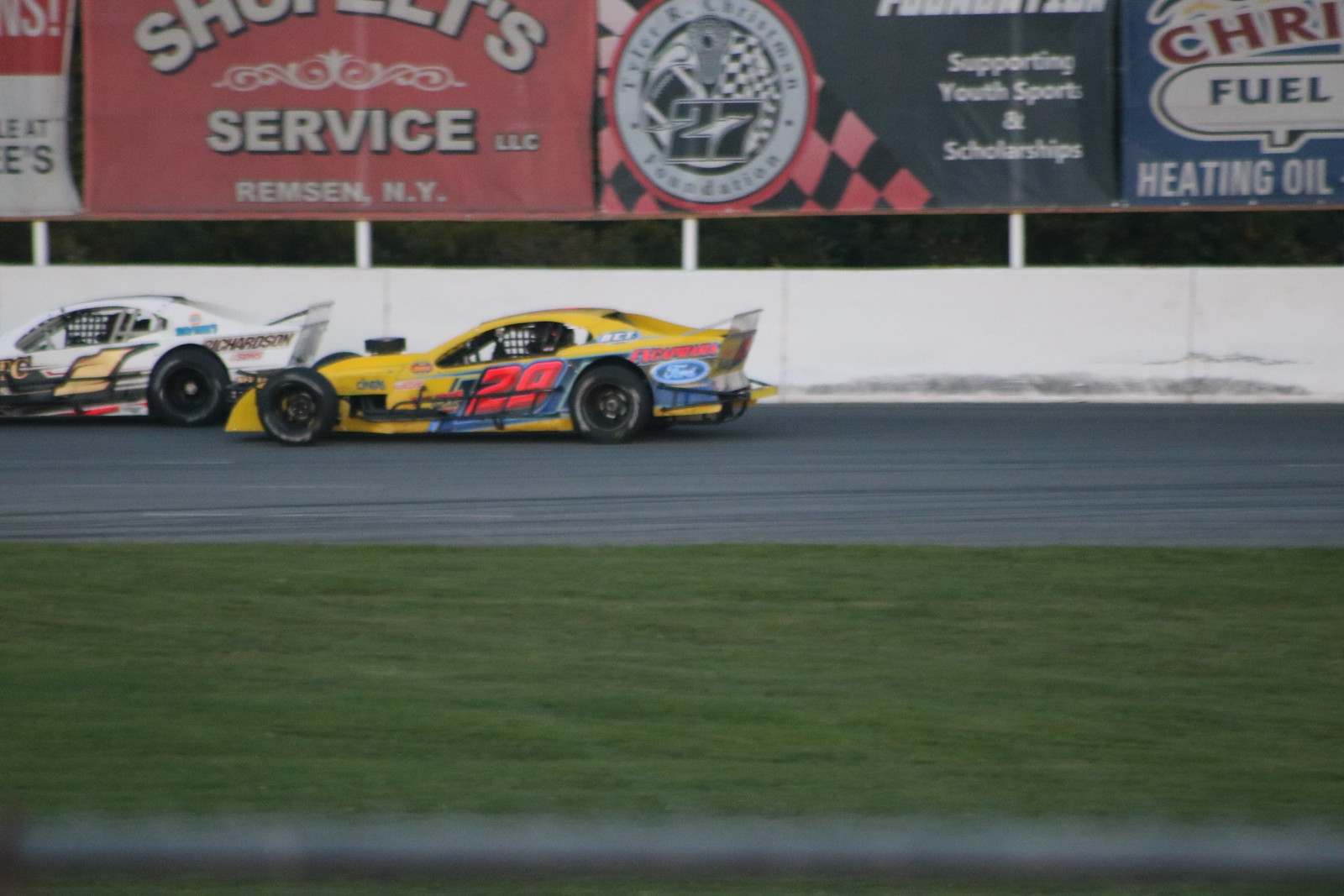A detailed photograph of a racing track captures two stock car race vehicles in action. Both cars are prominently displayed on the well-manicured green grass foreground of the track. The car in the front or to the left is a white vehicle featuring a gold number "1" on its side. Although difficult to distinguish, various small sponsor logos are also present. Behind it, or in the middle of the image, there's a striking yellow car marked with a red number "29" and a visible Ford logo on its rear quarter panel, indicating Ford sponsorship. The image also shows a barrier wall lined with advertisements or sponsorships, and a sign in the background reads "Service LLC," adding to the authentic racetrack environment.